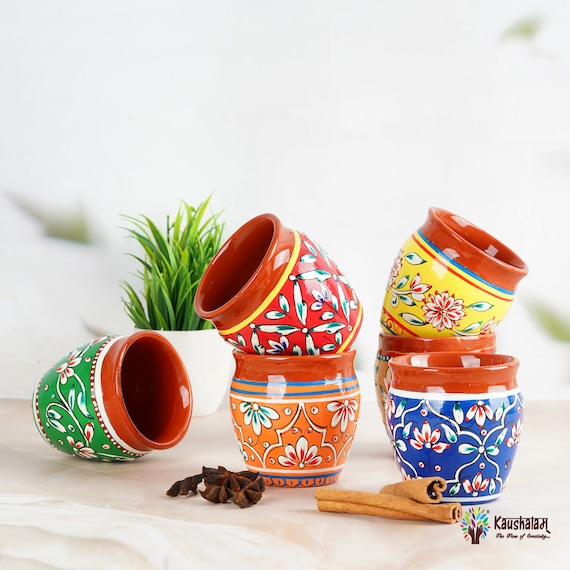The image showcases five small, ornate terracotta pots displayed on a pinkish tan and white marble countertop. Four of the pots are stacked in two separate piles, while one pot, featuring a green floral pattern on the bottom and a red terracotta neck, lies on its side with the opening facing right. The other pots display vibrant hues and floral designs: one is orange with a floral pattern, another is blue with flowers and bows, another is yellow with floral details, and a red pot with a similar floral motif completes the grouping. Each pot has a distinctive red-brown terracotta rim. Placed in front of the pots are sticks of cinnamon and small star anises. A blurred white background highlights a smaller white pot holding a green grass-like plant, contributing to the detailed and decorative nature of the scene. A hair scrunchie, seemingly balled up, can also be spotted on the table.